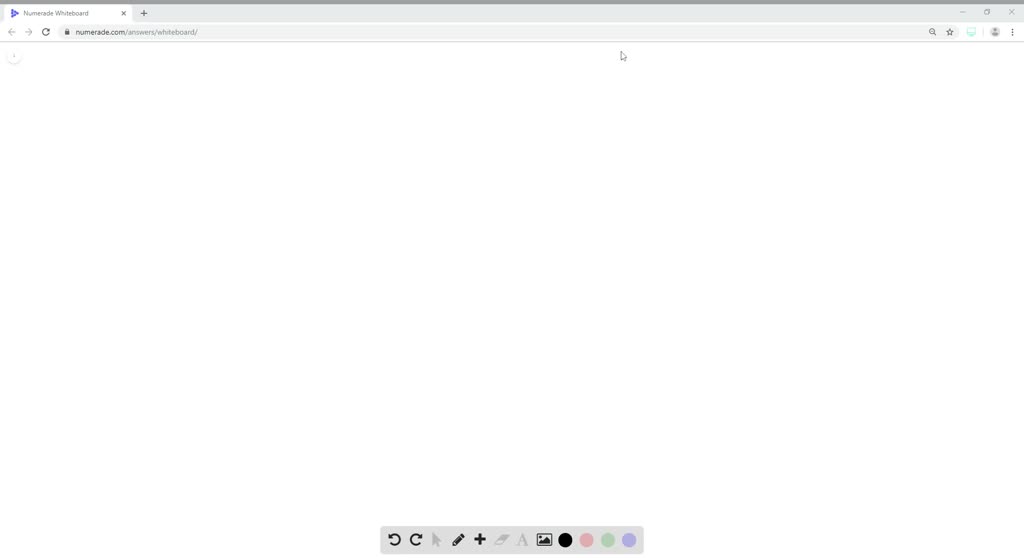Caption: 

A screenshot captures a computer screen displaying a web browser with an incomplete webpage load. The majority of the screen is blank white, indicating the page has not yet rendered. At the top, a thin gray bar shows minuscule text and numerical details, though they are too small to decipher. Below, a bottom toolbar is visible, featuring several buttons including 'Go Back,' 'Go Forward,' 'Edit,' 'Add,' and 'Image.' Among these, 'Go Back,' 'Go Forward,' 'Edit,' 'Add,' and 'Image' buttons are active, while the 'Font' button and several others remain unhighlighted. A distinctive black button with a circle is also present in the toolbar. The overall scene suggests the user is in the initial stages of navigating or editing a web page.